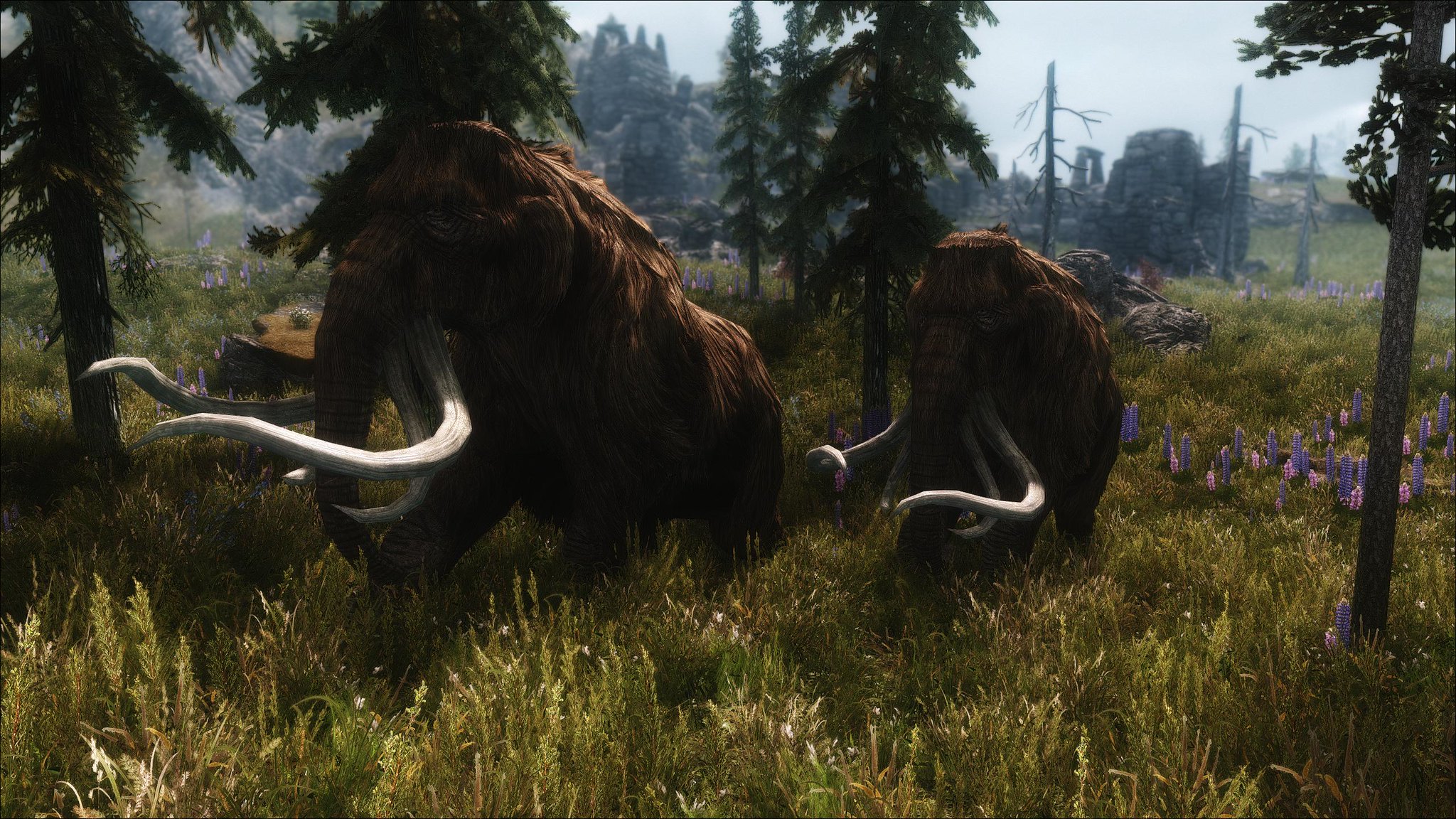This vividly detailed and fantastical scene, likely derived from AI-generated art or a video game like Skyrim, portrays two woolly mammoths traversing a verdant field of long, yellowish-green grass. The larger mammoth, positioned to the centre-left, is closely trailed by a smaller counterpart on the centre-right. Both animals exhibit dark, shaggy fur illuminated by an orangish-red rim light, giving them an almost ethereal glow. They also feature prominent, curved white tusks—two large and two smaller secondary tusks on each mammoth. Their faces are obscured in shadow, emphasizing the grandeur of their looming tusks and towering frames.

The backdrop is a lush landscape punctuated by tall, slender trees reminiscent of firs, alongside a cluster of dark-leafed, long-trunked trees. A striking horizontal row of purple flowers, akin to bluebells or hyacinths, enhances the scenery to the right, behind the smaller mammoth. The distant background reveals a grey sky and hints of tall mountains, adding depth to the scene. Moreover, there seems to be a suggestion of ancient human ruins or a fortress, invoking a sense of timeless mystery and adventure, as if part of a grand, untouched world.